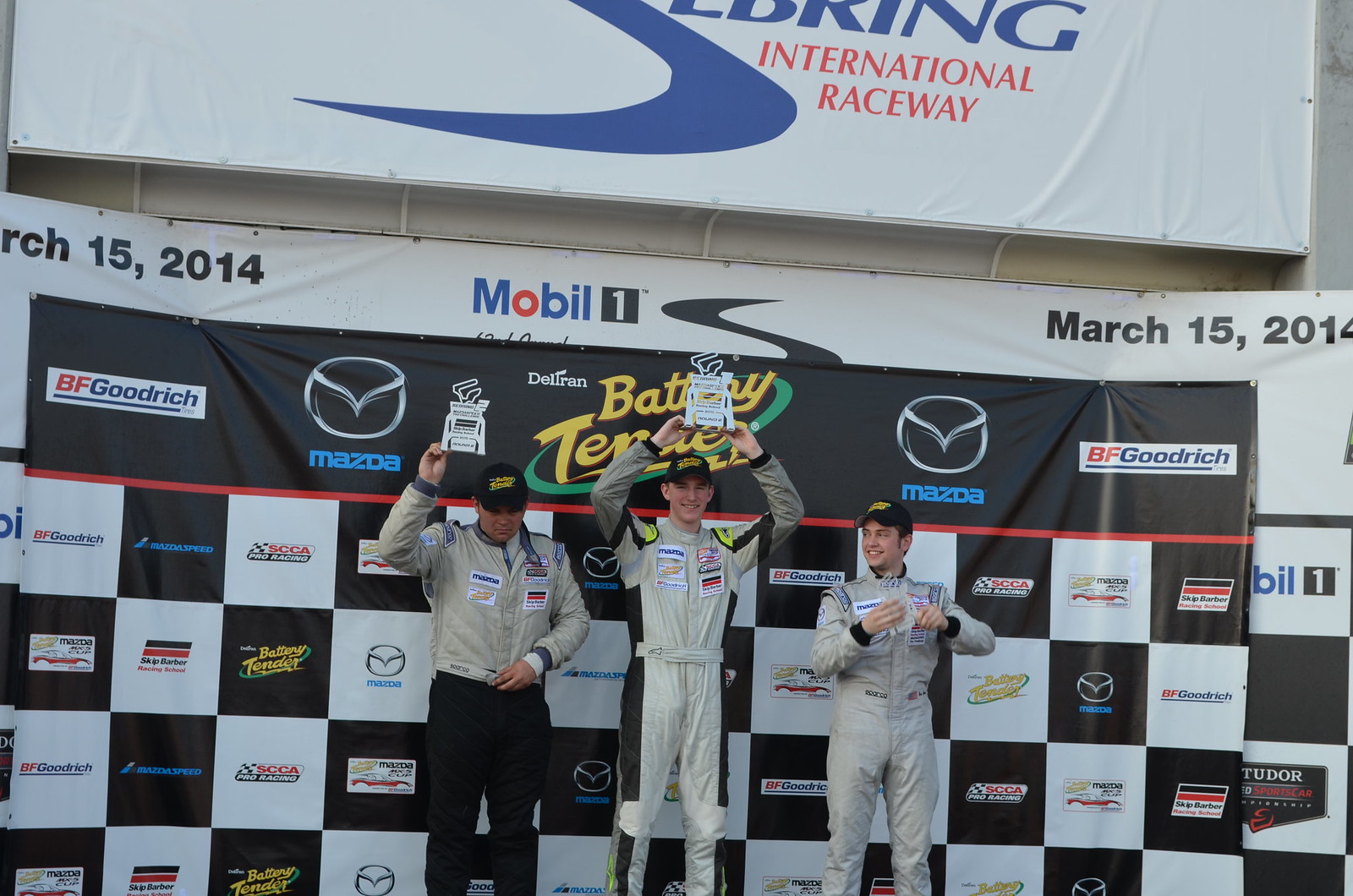In the winner's circle at Sebring International Raceway, beneath a prominent sign reading "Sebring International Raceway" and a date banner indicating March 15, 2014, three victorious men stand shoulder to shoulder, proudly displaying their trophies. The man in the center, wearing a full light gray racing uniform adorned with chest patches, triumphantly holds a white trophy with a chrome-colored wire accent above his head. His black hat, featuring orange writing, stands out against his outfit. To his left, a man in a light gray jacket and black pants raises his trophy high with one hand while resting his other hand in front of his stomach. The man on the right, clad in a solid gray racing suit and a black hat, smiles slightly as he holds his trophy in front of his chest, turning his face to the right. Behind them stretches a checkerboard backdrop filled with advertisements, prominently featuring brands like B.F. Goodrich and Mazda. A long black banner boldly displays "B.F. Goodrich" and "Mazda" branding, while a partially obscured advertisement with the word "battery" in yellow lettering hints at its presence. Above all, a white banner with red letters announces the "International Raceway," capturing the spirit and excitement of the moment.